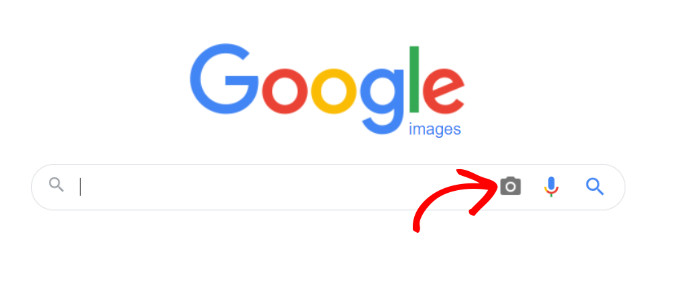This image depicts a very plain, minimalistic interface with a white, rectangular background. Dominating the top portion, it features the Google logo in large, colorful letters: the two G’s are blue, the first O and the E are red, the second O is yellow, and the L is green. Directly below the Google logo, aligned towards the right and under the L and E, the word "Images" appears in small blue text.

Stretching horizontally across the page, a prominent search bar takes center stage. On the left end of the search bar, there's a small gray magnifying glass icon. Adjacent to this icon, a thin vertical line separates it from the rest of the search bar. A hand-drawn red arrow directs attention towards the camera icon situated on the right side of the search bar. Beside the camera icon, another icon depicts a microphone.

On the far right end of the search bar, a larger blue magnifying glass icon mirrors the smaller gray one on the left. The simplicity is striking, with no additional text, photos, or artwork, emphasizing the clean, uncluttered design.